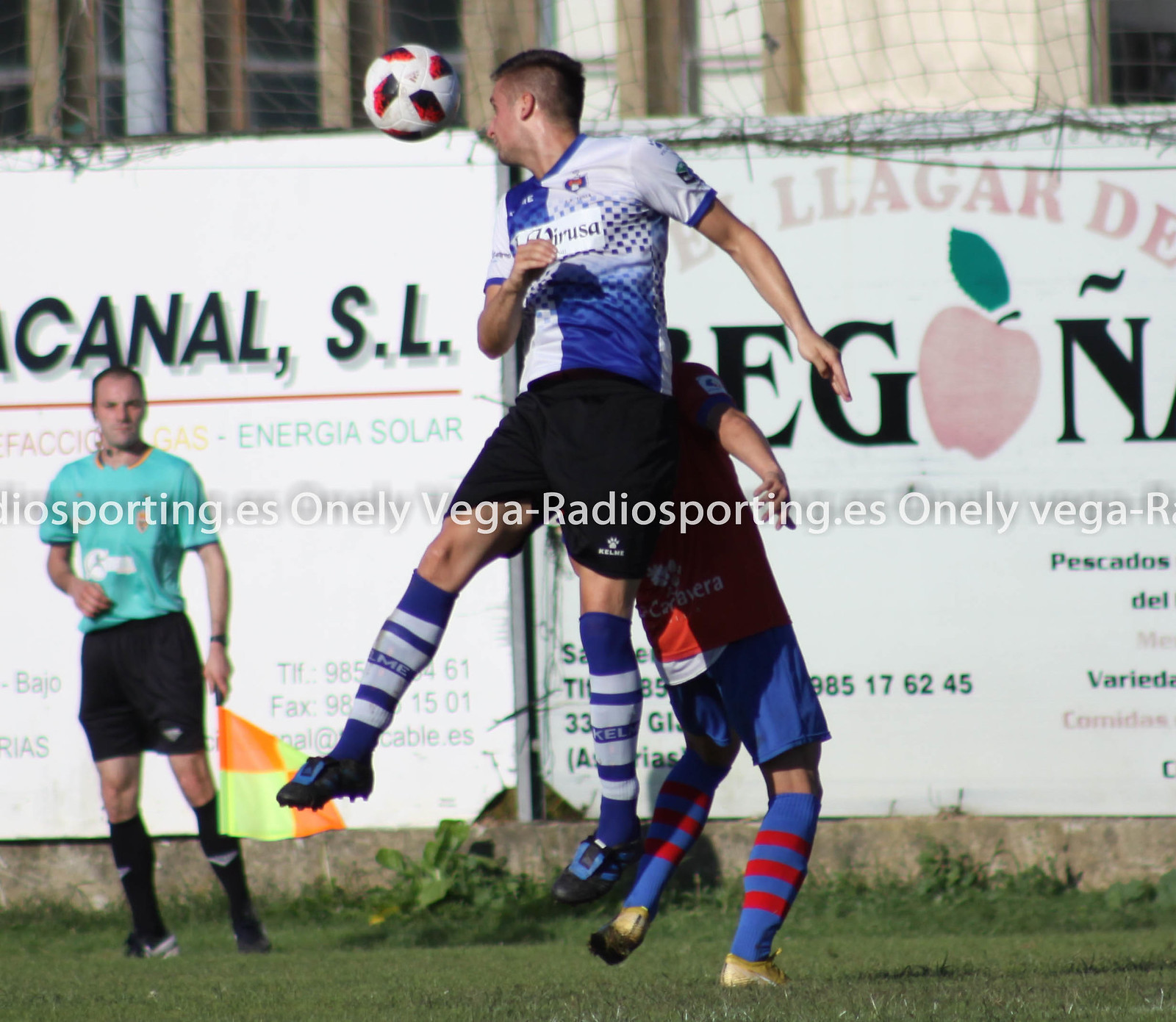In a vibrant snapshot of a soccer match, two players fiercely contest the ball, capturing the intensity of the game. In the foreground, one player, clad in a mix of blue and white jersey, leaps into the air, his head turned to his left as he aims to hit the predominantly white soccer ball, marked with red and black patterns. He sports blue and white striped shin guards. His opponent, slightly hunched back from the impact, wears a darker blue or black jersey, paired with dark blue pants and blue and red-striped shin guards. To the left, a referee is pictured in a light blue shirt, black shorts, and black shin guards. His left arm rests near his waist, while his right hand holds a distinctive flag with orange and yellow quadrants. In the background, advertising billboards with the text "Canal SL" and an Apple company logo add to the authenticity of the sporting event.